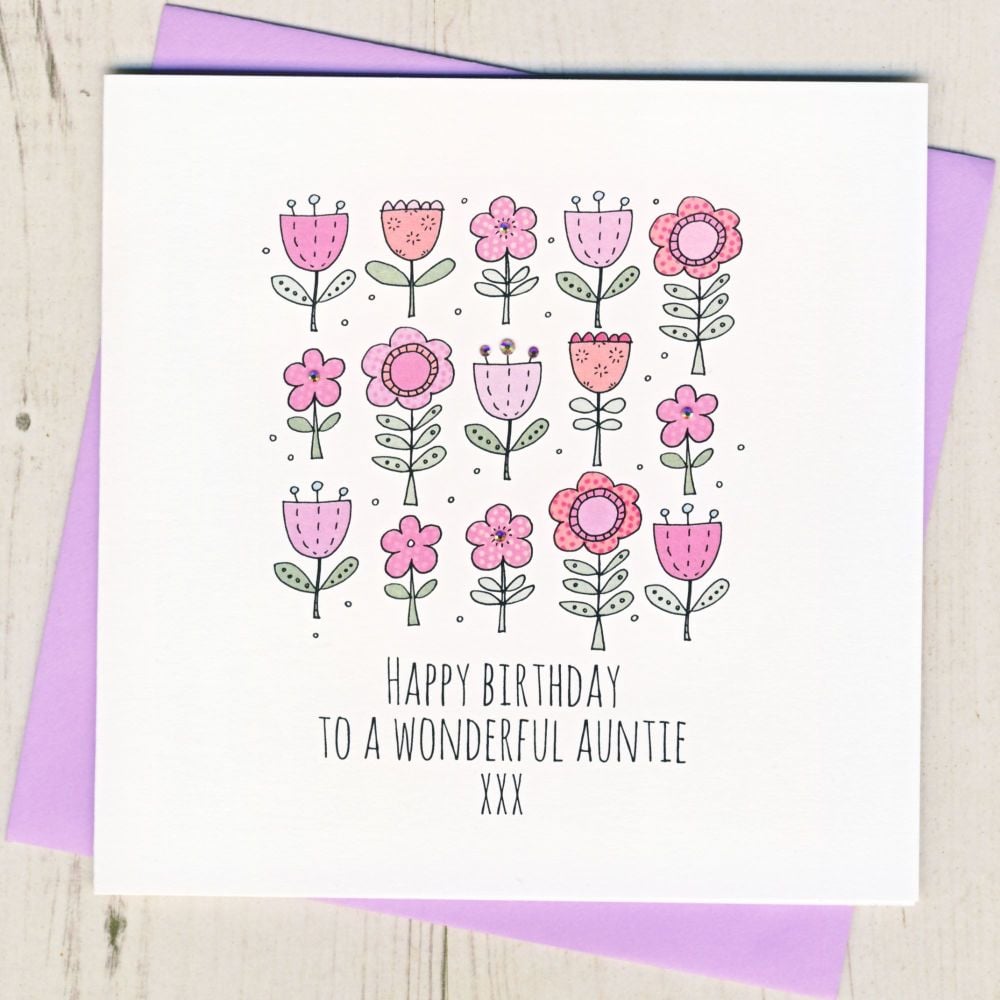This image depicts a “Happy Birthday to a Wonderful Auntie” card sitting on a light beige wooden surface. The white greeting card features an artistic arrangement of five rows of flowers, each containing a variety of tulips and other blossoms depicted in shades of pink, peach, and purple. Each flower is outlined in black, with some containing decorative geometric shapes and others having traditional petal designs. The bottom of the card displays the phrase "Happy Birthday to a Wonderful Auntie xxx" in thin black lettering. A purple envelope, partially visible and slightly angled to the right, matches the purple hues in some of the flowers, adding a cohesive touch to the arrangement.